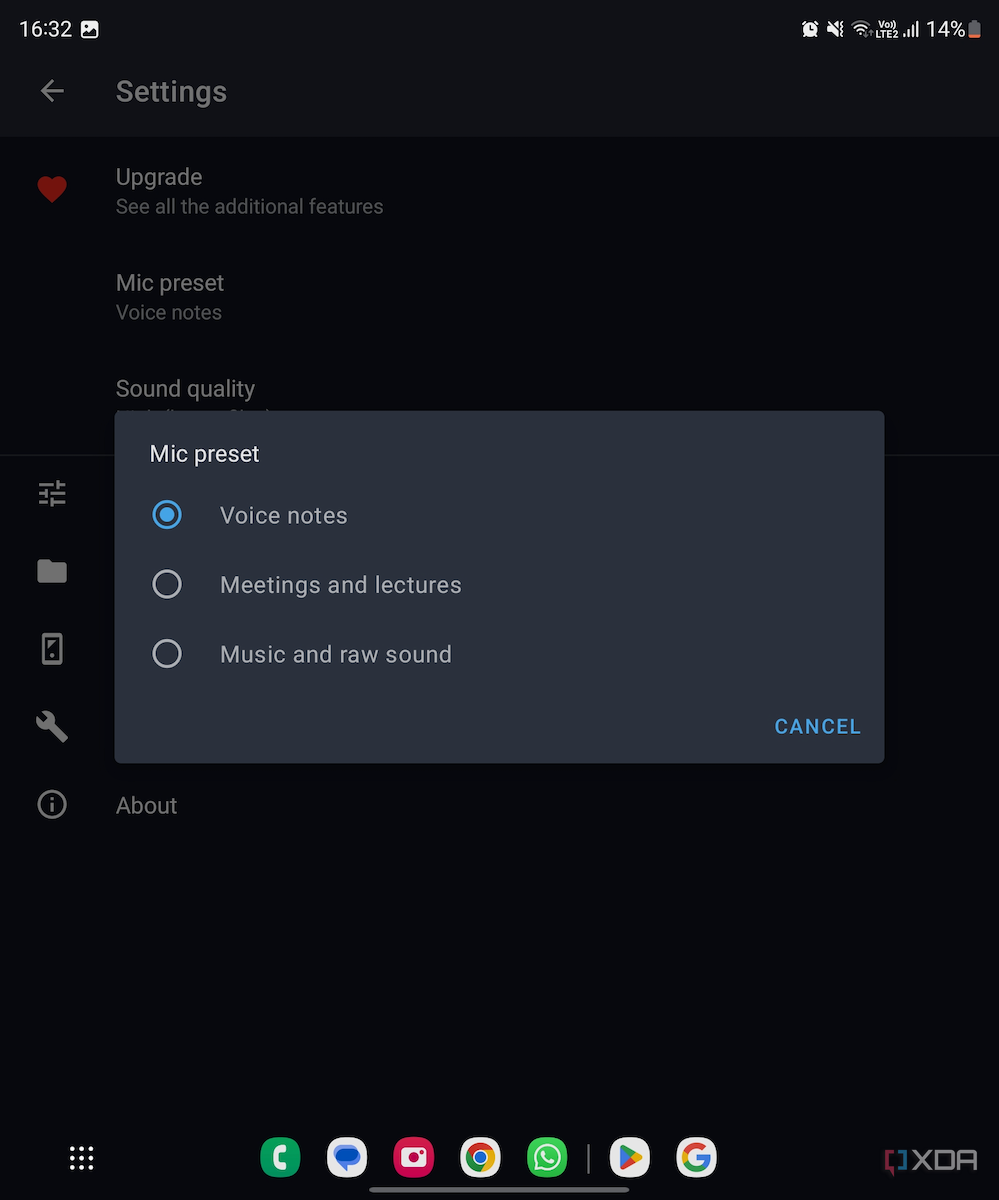The image depicts a smartphone interface set against a black background. At the top of the screen, the time is shown as 16:32 along with an alarm clock icon. The battery level is displayed at 14%, accompanied by a battery icon. 

A settings icon and a left-pointing arrow are also visible at the top. Below these elements, the interface features an “Upgrade” prompt, encouraging users to “see all the additional features,” highlighted with a red heart symbol.

Central to the screen are several mic presets listed under categories such as "Voice Notes," "Meetings," and "Featured Lectures." The "Voice Notes" option is emphasized with a blue highlight. Adjacent to these options are three radio dial buttons.

At the bottom of the screen, a blue "Cancel" button is presented. Additionally, there is a grid of icons organized in three rows of three white squares. These include symbols for phone calls, chats (chat icon), a camera, Google Chrome, WhatsApp, Google Music (depicted as a triangle in Google colors), and the Google app (represented by a "G" in Google colors).